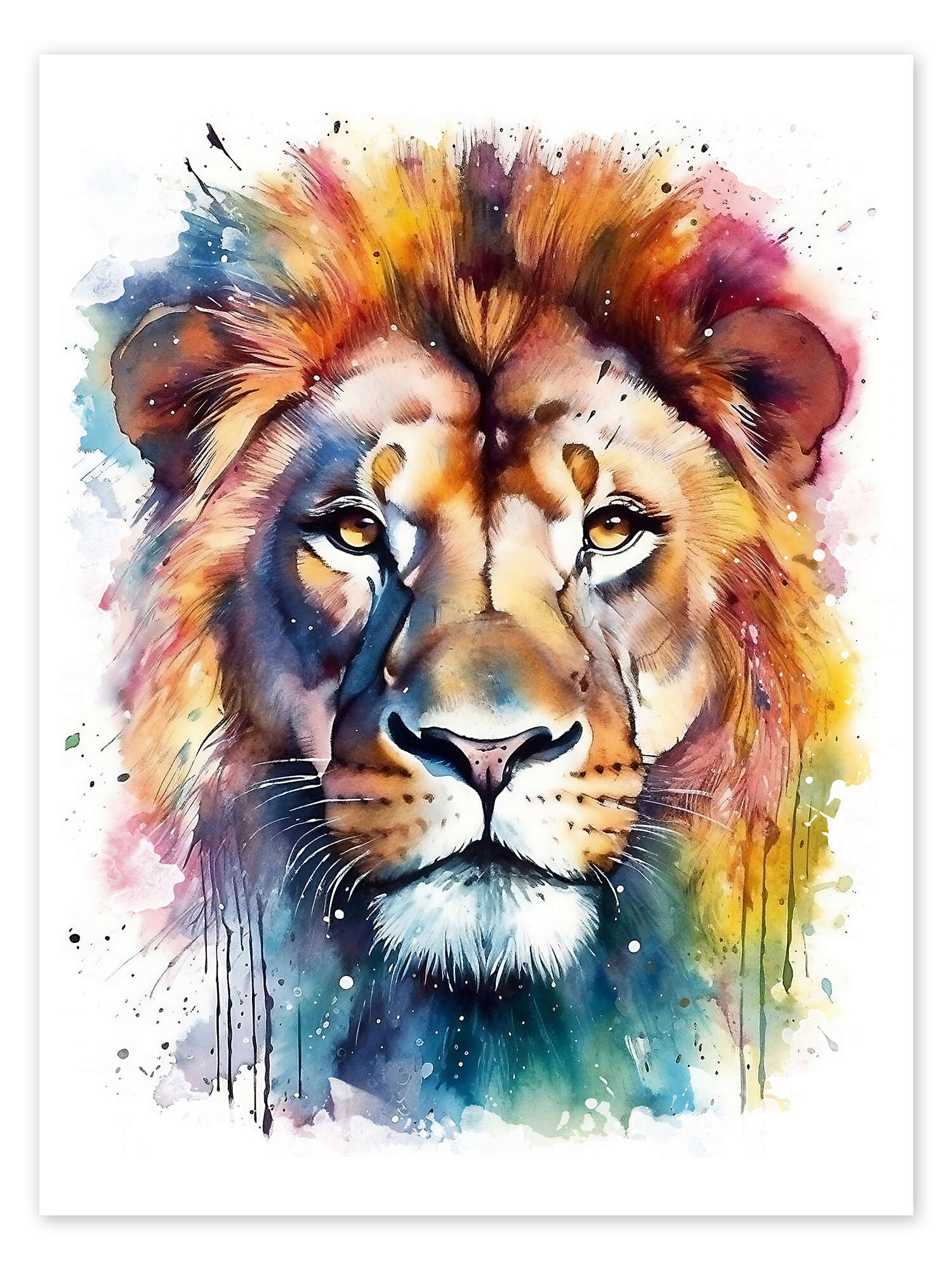This is a stunning and vivid painting of a lion’s head, facing straight at the viewer, set against a crisp white background. The artwork is done in a watercolor style, featuring a kaleidoscope of colors including shades of purple, orange, brown, yellow, red, pink, and blue. The lion's eyes are predominantly yellow with hints of green, giving a deep, piercing gaze. The fur is depicted using splotchy and splattered paint techniques, with small dots indicating the splatters. Muted tones like deep pink, plum, and a muted blue also highlight the lion's fur. The lion has small, round ears, and whiskers visible near the mouth. Overall, the portrait suggests a determined expression and captures the majestic essence of the lion in a beautiful and artistic manner.